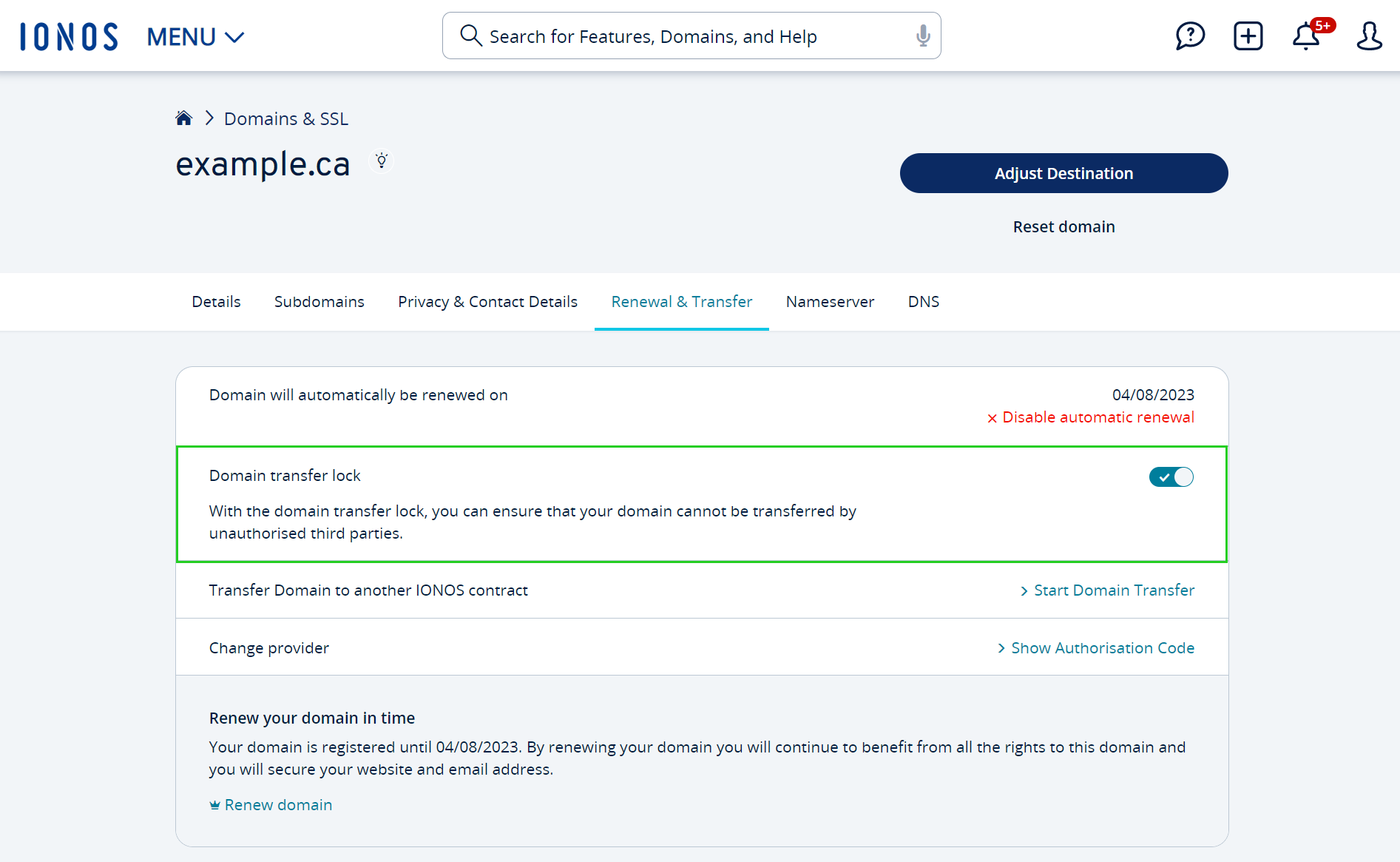The screenshot depicts a webpage with a structured header and a partially visible body section. The header is predominantly white and consists of several key elements, beginning with a blue logo labeled "Ionis." The design of the "N" in "Ionis" incorporates artistic white lines that mirror the angle of the slanted line within the letter. 

Adjacent to the logo is the word "MENU" in bold, uppercase blue text, which is followed by a downward-pointing blue arrow. To the right of ample spacing, a search bar is visible, characterized by its white background, thin light gray outline, and gently rounded corners. The left side of the search bar features a gray magnifying glass icon, while the right side has a light gray microphone icon. The placeholder text within the search bar reads "Search for features, domains, and help" in gray font.

Further to the right, separated by more negative space, there are four distinct black icons: a speech bubble with a question mark inside, a square with rounded corners and a plus sign, a bell adorned with a red notification indicator displaying "5+", and a profile picture icon.

Beneath the header, the body section of the page appears against a very light blue background. A subtle medium gray shadow delineates the boundary between the header and the body. In the upper left corner of the body, a dark blue home icon is followed by a right-pointing arrow and blue text that says "Domains and SSL." Directly below this, prominent large black text displays "example.ca," with a small blue lightning bolt icon featuring three dots along its top, situated to the right.